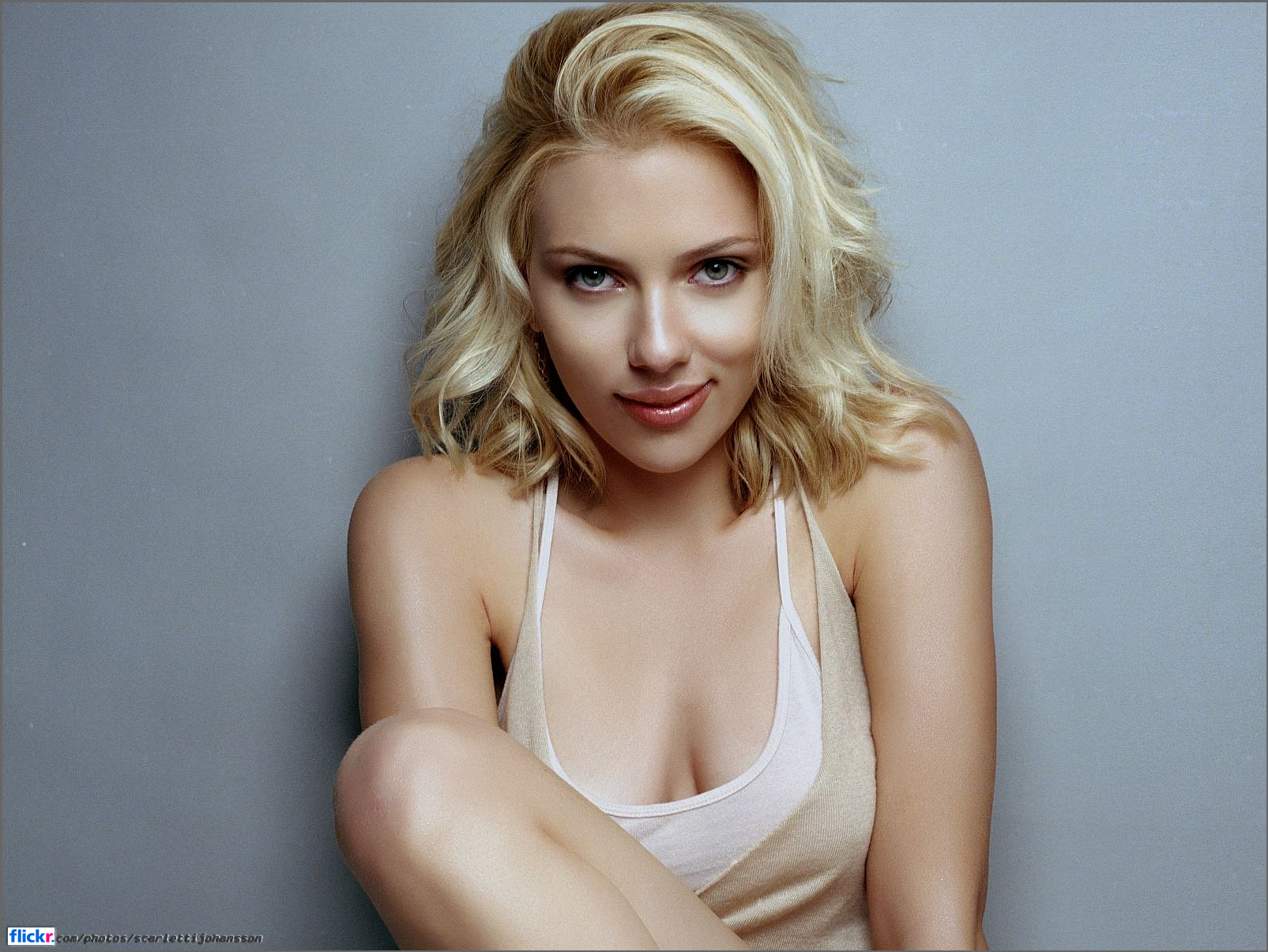This photo is a posed portrait of Scarlett Johansson, seated against a solid gray background. She is captured from the waist up, with her bent leg and knee prominently visible, partially covering her torso. Scarlett is wearing a low-cut white tank top with spaghetti straps, layered beneath an even lower beige tank top. Her tousled, windblown blonde hair sweeps over to the right side of her face, while some strands hang down below her shoulders. Her lips are accentuated with reddish-pink lipstick, and she gazes directly at the camera. At the bottom left of the image, a URL reads flickr.com/photos/ScarlettJohansson, accompanied by the Flickr logo.